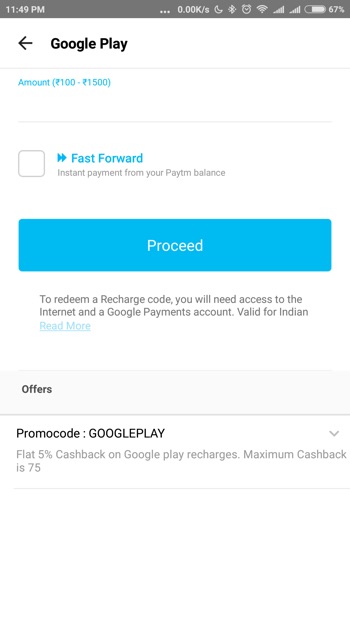The image features a detailed interface of a mobile screen, displaying a Google Play recharge process with an array of information and status icons. At the top, against a gray background, white text reads "11:49 PM." Next to it, there are three dots followed by "0.0 K/s." To the right, icons depict a crescent moon (likely indicating night mode), GPS, a clock, full Wi-Fi signal, two full bars of cell service, and a battery icon that is approximately 25% full, indicating 67% battery remaining.

The main content area has a white background with black text. A left-pointing arrow is labeled "Google Play," followed by a grayscale loading bar moving left to right. Beneath this bar, in blue text, the word "Amount" appears, succeeded by a quoted text: "₹100 to ₹1,500." Another green line is present below.

On the left-hand side, a small blue square icon is shown. To the right, are two buttons labeled "Fast Forward," suggesting instant payment options from the user's Paytm balance. The language "instant payment from your Paytm balance" appears underneath.

Dominating the lower part of the screen is a large blue button with the word "Proceed" centered in white. Below this button, gray text indicates that to redeem a recharge code, internet access and a Google Payments account are needed. It further notes that this service is valid only for India. To the left-hand side, an underlined blue text reads "Read More."

Towards the bottom, in a gray-shaded section with black text, the word "Offers" stands out. Below, in a white section with black text, a promotion is detailed: "Promo Code Google Play." This is accompanied by gray text explaining the promo, "Flat 5% cashback on Google Play recharges, maximum cashback is ₹75."